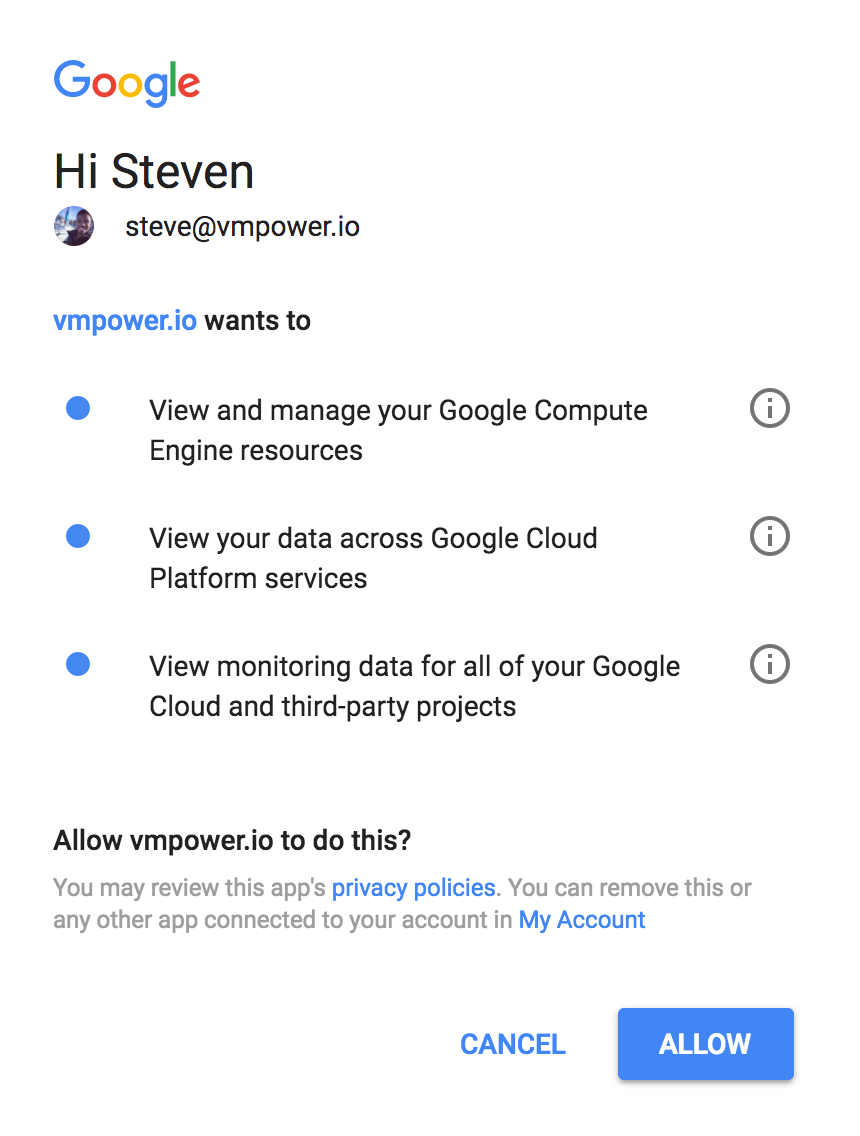The image shows a Google authorization prompt featuring the company's iconic logo in the top left corner, which includes a blue capital 'G', followed by the letters in red, yellow, blue, green, and red, spelling out "Google." Below this, in black text, it reads "Hi Steven," alongside a circular avatar featuring Steven's picture. To the right, it lists "steve@vmpower.io" followed by "vmpower.io" in blue text. 

The prompt below it states in black, "wants to," followed by three bulleted permissions in blue:
1. "View and manage your Google Compute Engine resources," accompanied by a gray circle with a lowercase 'i' inside.
2. "View your data across Google Cloud platform services," also marked with a similar gray circle containing a lowercase 'i'.
3. "View monitoring data for all of your Google Cloud and third-party projects," again noted with a gray circle featuring a lowercase 'i'.

Underneath, it asks in black text, "Allow vmpower.io to do this? You may review this app's privacy policies. You can remove this or any other app connected to your account in My Account." Finally, at the bottom, there are two action buttons: one saying "CANCEL" in blue capital letters, and another blue rectangular button labeled "ALLOW" in white capital letters.